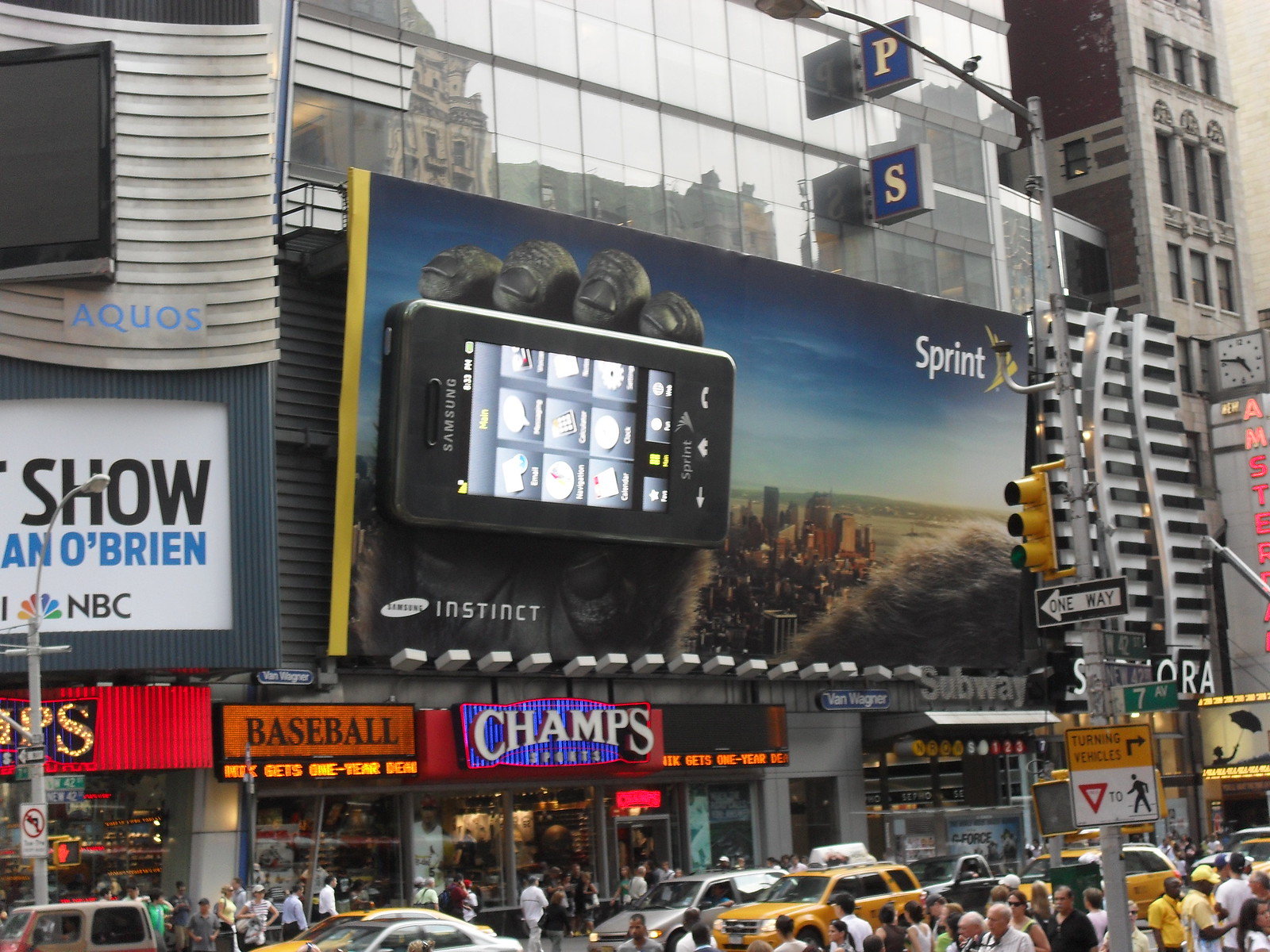In this photograph taken in a bustling urban city, the focus is on a large rectangular billboard prominently displayed on the glass-paneled side of a skyscraper. The billboard features a striking image of a monkey hand gripping a large, flat smartphone adorned with silver text that reads "Samsung." The billboard's background showcases an aerial view of a cityscape. In the top right corner of the billboard, the logo and name "Sprint" are clearly visible in white text.

Below the billboard, positioned along its bottom edge, are several square-shaped white spotlights aimed upwards, currently turned off due to the daylight. Beneath the towering structures and the billboard, the lower section of the image captures the street level, where a plethora of pedestrians and vehicles are stuck in traffic, adding to the vibrant and dynamic atmosphere of the city. The photograph, rectangular in shape with the top and bottom sides longer than the left and right sides, adeptly captures the essence of urban life and modern advertising.